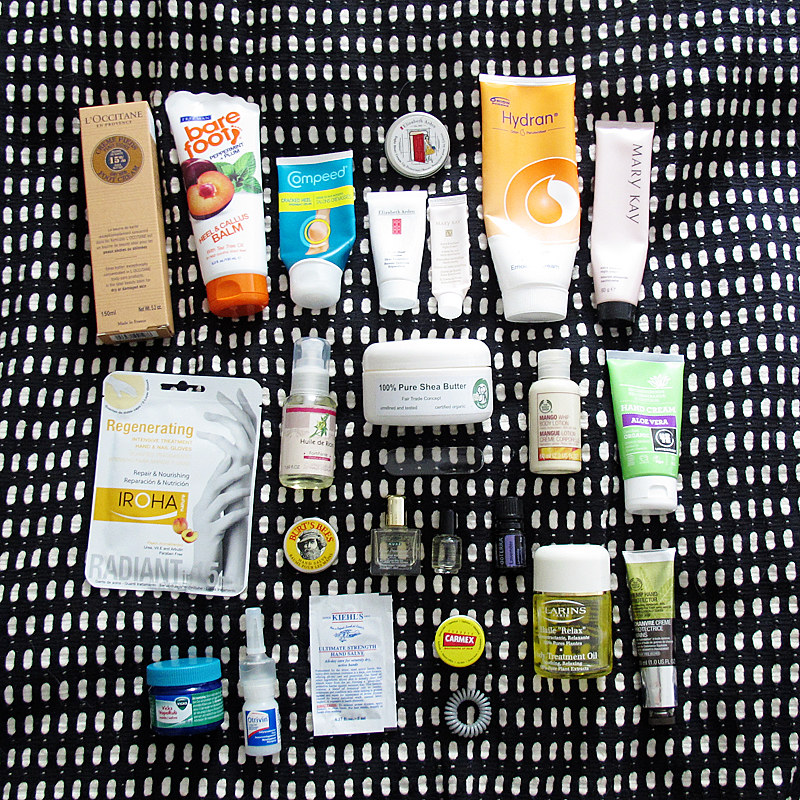The image features a collection of foot and nail care products arranged neatly on a black and white grid-patterned cloth. The items are organized in three to four rows. Starting from the top row, the first product is a rectangular brown package from L'Occitane. Next to it is a tube labeled "Barefoot," which is a callus balm. Among the products are various nail polishes, tubes, and tubs. In the middle row, there's a white tub with a white lid labeled "100% Pure Shea Butter." At the bottom right, there's a tube of nail cream. On the bottom left, there's a product that resembles a Vicks item. Additionally, one of the items is a Burt's Bees product in a lip balm form. Lastly, on the top right, there's a product from Mary Kay. The assortment includes both skin care and nail care products, ranging from balms and creams to polishes and treatments.